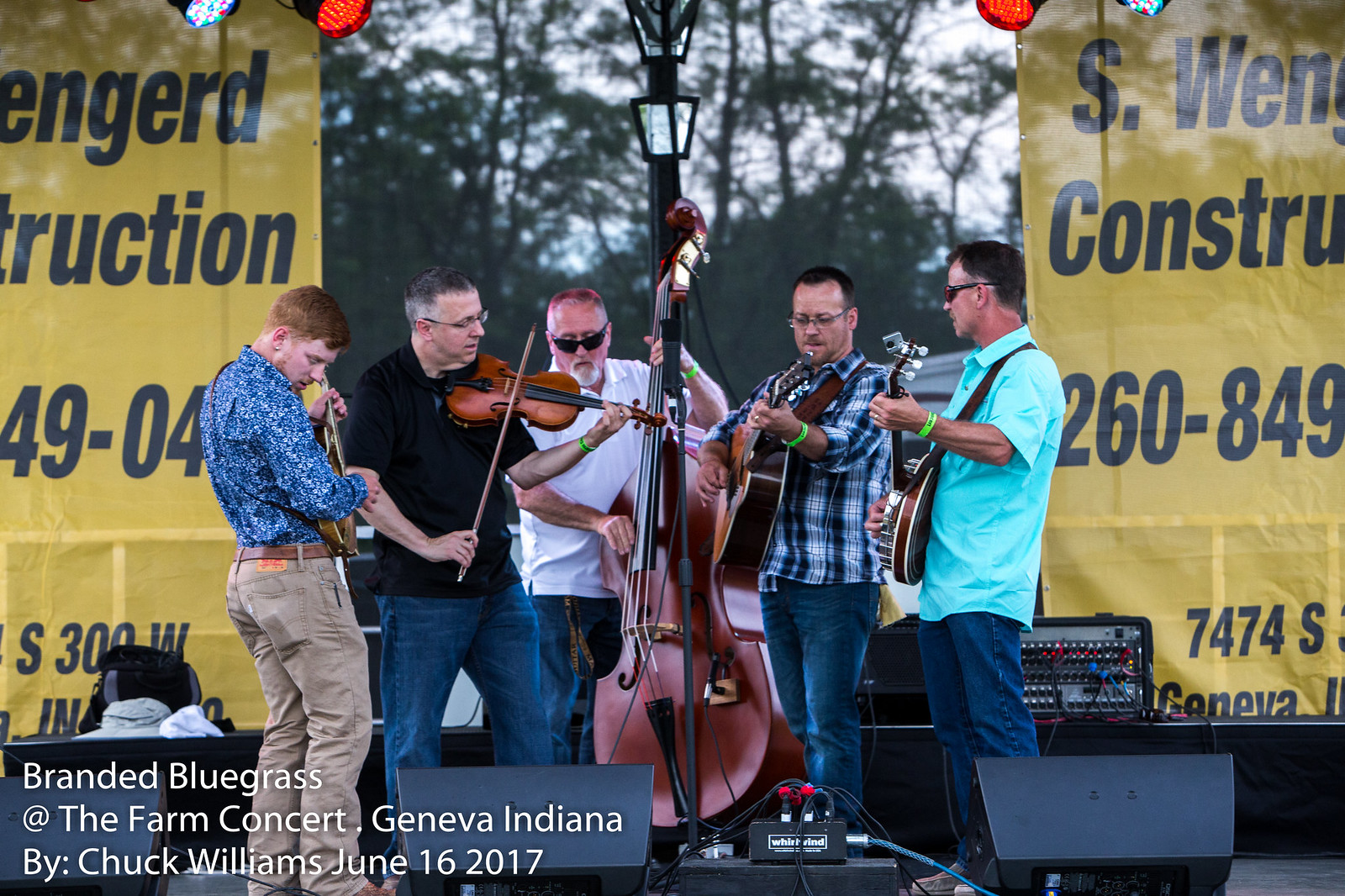This image captures an outdoor performance by the five-member band "Branded Bluegrass" at the Farm Concert in Geneva, Indiana, on June 16, 2017, photographed by Chuck Williams. The band members, all Caucasian males, range in age from a redhead in his 30s to others who appear to be in their 40s or older. They are dressed casually in sports shirts and jeans, with two wearing sunglasses. The ensemble features a variety of musical instruments, including acoustic guitars, a violin, a banjo, and a string bass, set against a backdrop of trees and a lamppost. The stage is equipped with electronics, including a microphone and a speaker. Large yellow banners advertising "S. Wengard Construction" flank the stage, along with other indistinct promotional signs displaying telephone numbers. The caption in the lower left corner of the image reads: "Branded Bluegrass, The Farm Concert, Geneva, Indiana by Chuck Williams, June 16, 2017."